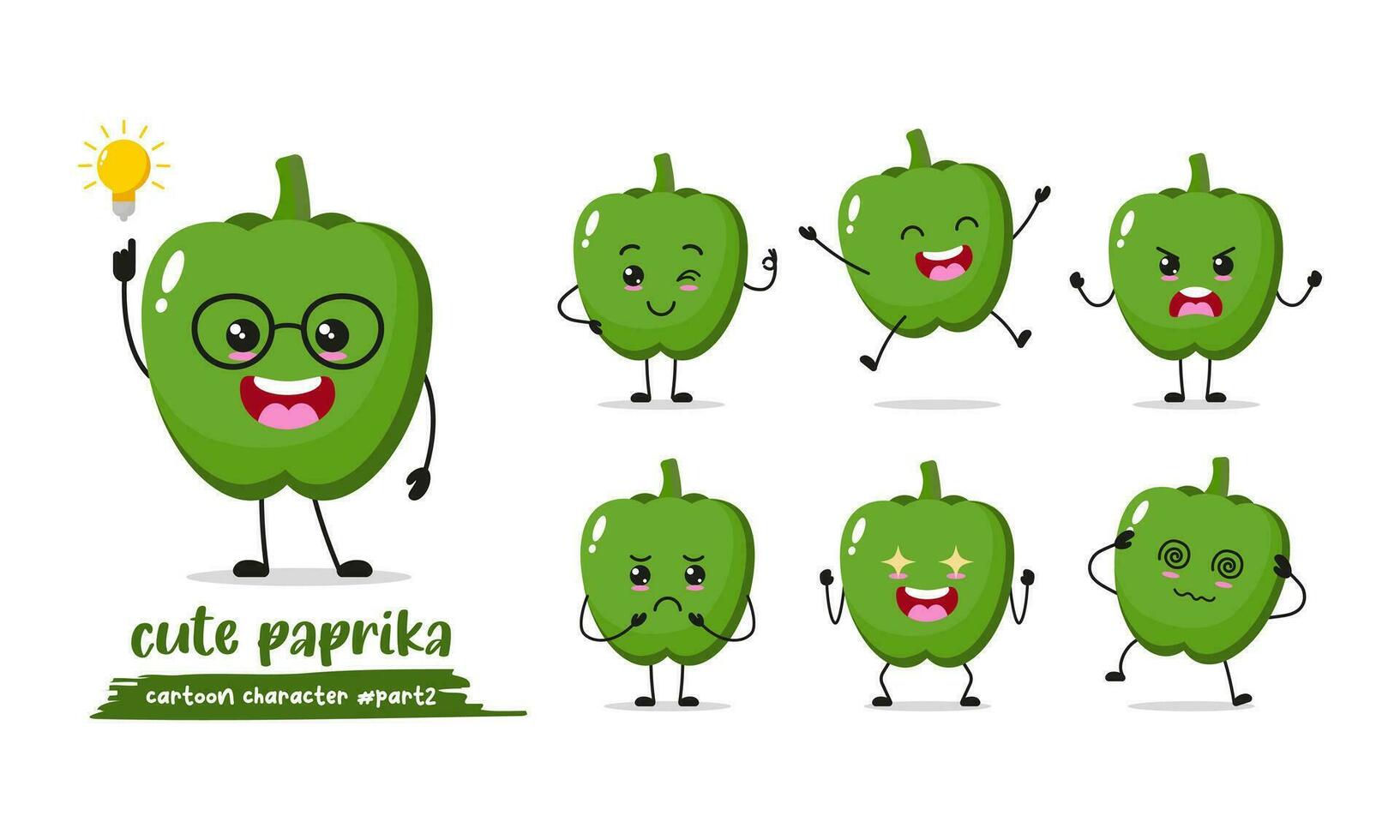This image is a color slide depicting a collection of green peppers, arranged in a lively, cartoonish manner. The focal point is a large green pepper located on the left side of the image, designed with human-like features including eyes, a mouth, arms, and legs. It wears little black glasses and appears to be pointing up towards a yellow light bulb. Below this character are the words "Cute Paprika Cartoon Character Part 2." 

To the right of this central figure are six smaller green peppers, each displaying a unique expression. The first pepper is winking one eye, while the second is jumping up in the air with excitement. The third pepper appears angry, the fourth looks sad, and the fifth has stars in its eyes with an open mouth indicative of pure joy. The final pepper has whirlpool eyes, is holding its head in its hands, and seems to be dizzy or confused. All the peppers have stems on top of their heads and sport simple black arms and legs, giving them a stick-figure-like appearance.